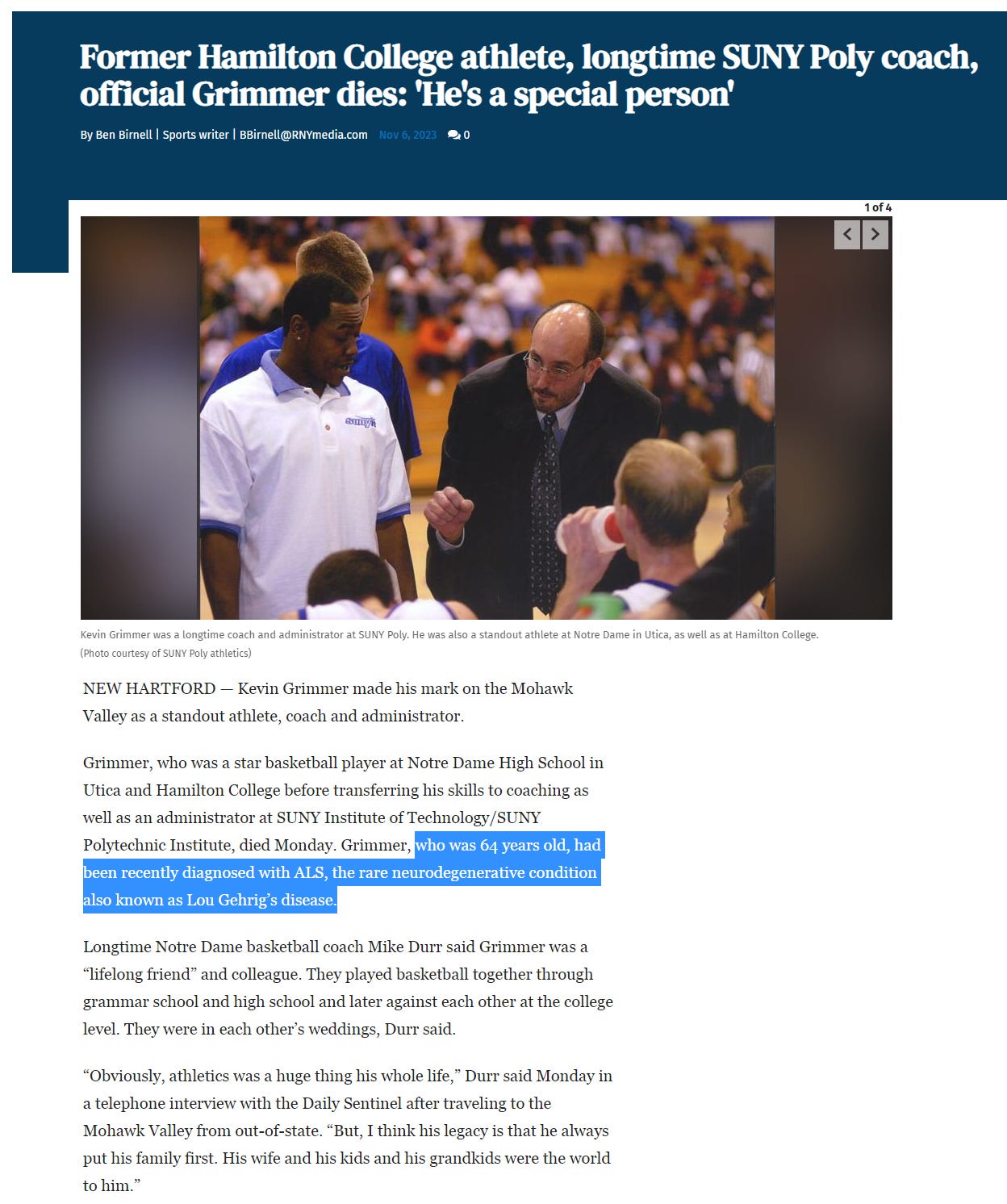This image is a screenshot of an online article. At the top, there is a prominent headline displayed against a blue banner, with the text presented in white. Immediately below the headline is the byline. The article is set against a clean white background with black text, except for one sentence in the first main paragraph, which is highlighted in blue.

A photograph is embedded within the text, depicting a middle-aged white man dressed in a suit. He has glasses, a beard, and a receding hairline. He appears slightly bent over as he engages in conversation with a group of student basketball players. To his right, other staff members are visible, suggesting a collaborative or supportive environment.

The highlighted sentence reads, "Grimmer, who is 64 years old, had been recently diagnosed with ALS, the rare neurodegenerative condition also known as Lou Gehrig's disease." The article continues with additional paragraphs providing further context and information.